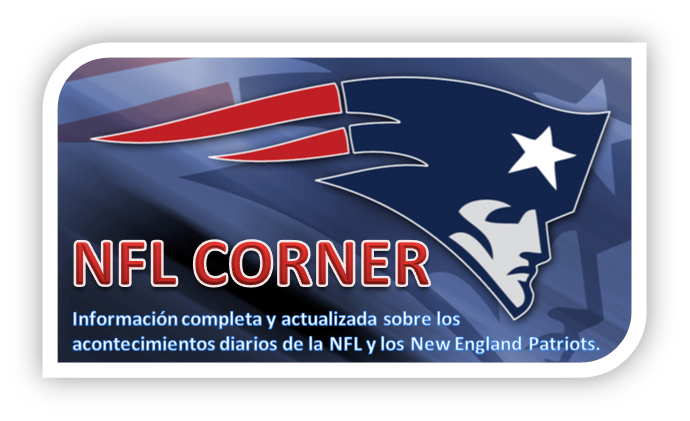The image features a rectangular design with rounded and pointed corners, enclosed in a white border. Dominating the left side of the blue background, "NFL Corner" is prominently displayed in red, all capital letters with a white outline. Below this, the text "Información Completa y Actualizada sobre los acontecimientos de la NFL y los New England Patriots" is written in Spanish, providing comprehensive and up-to-date information about the NFL and the New England Patriots. Positioned at the top right, the New England Patriots logo—depicting a side view of a Patriot with a dark navy-blue hat, a white star, and trailing red streamers—stands out. This logo partially overlaps onto the left side. The blue background also features a muted, outlined replica of the Patriots logo, adding depth to the design.